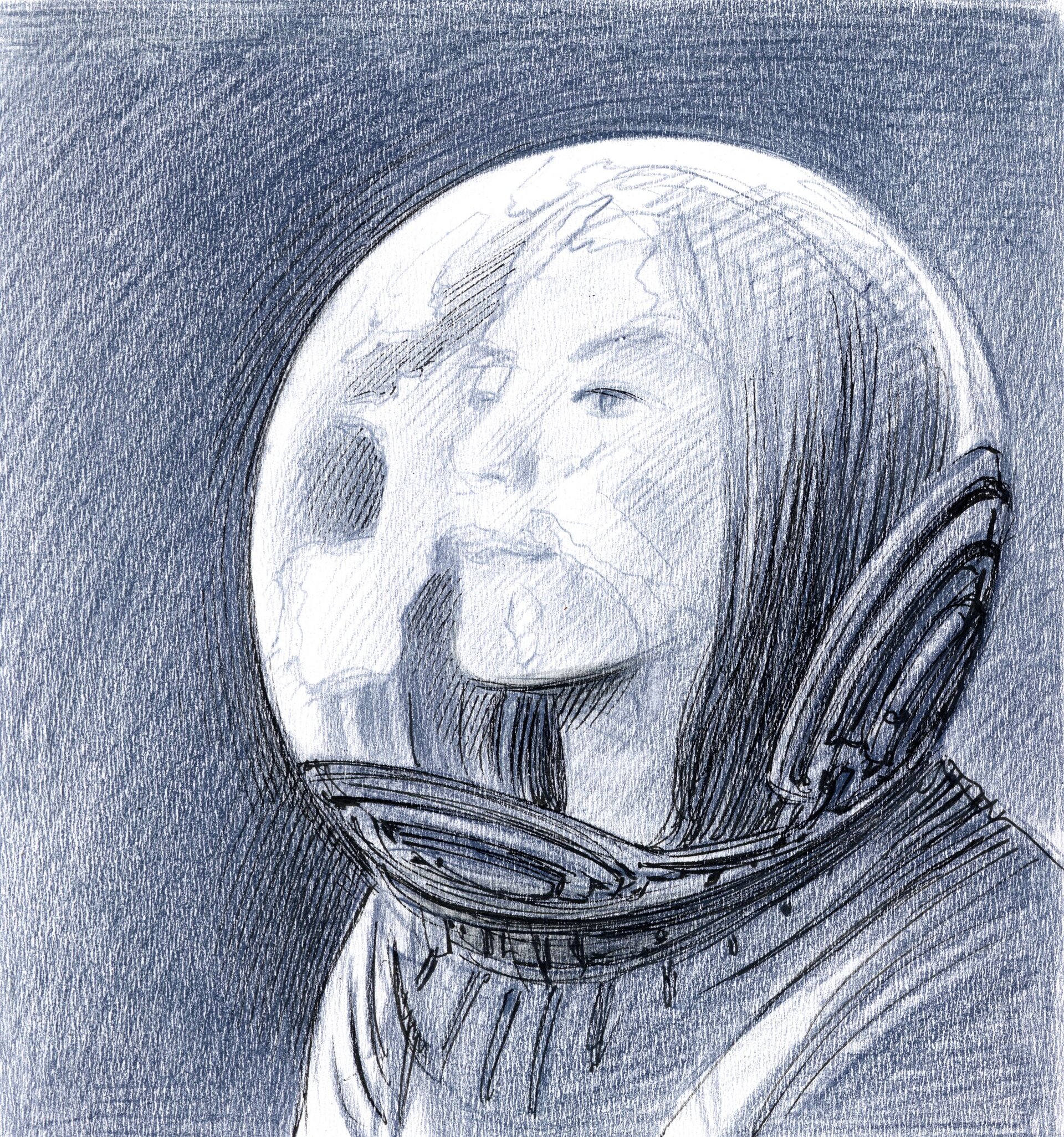The image is a detailed blue pencil sketch of a woman in a space suit, featuring a complete glass dome helmet with metal bracing at the front and sides, connecting to a ring structure attached to the suit. The woman, who appears to be white with long, dark hair and a strong, jutting chin, is well-lit with her face illuminated, showing one eye, an eyebrow, and her nose in profile. Her calm, pensive expression includes a slight smirk as she looks diagonally to the left, seemingly back at planet Earth, which is faintly reflected in her helmet. The suit includes intricate detailing, characteristic of a typical bulky astronaut suit, contrasting with the dark, cross-hatched background that lightens at the edges.